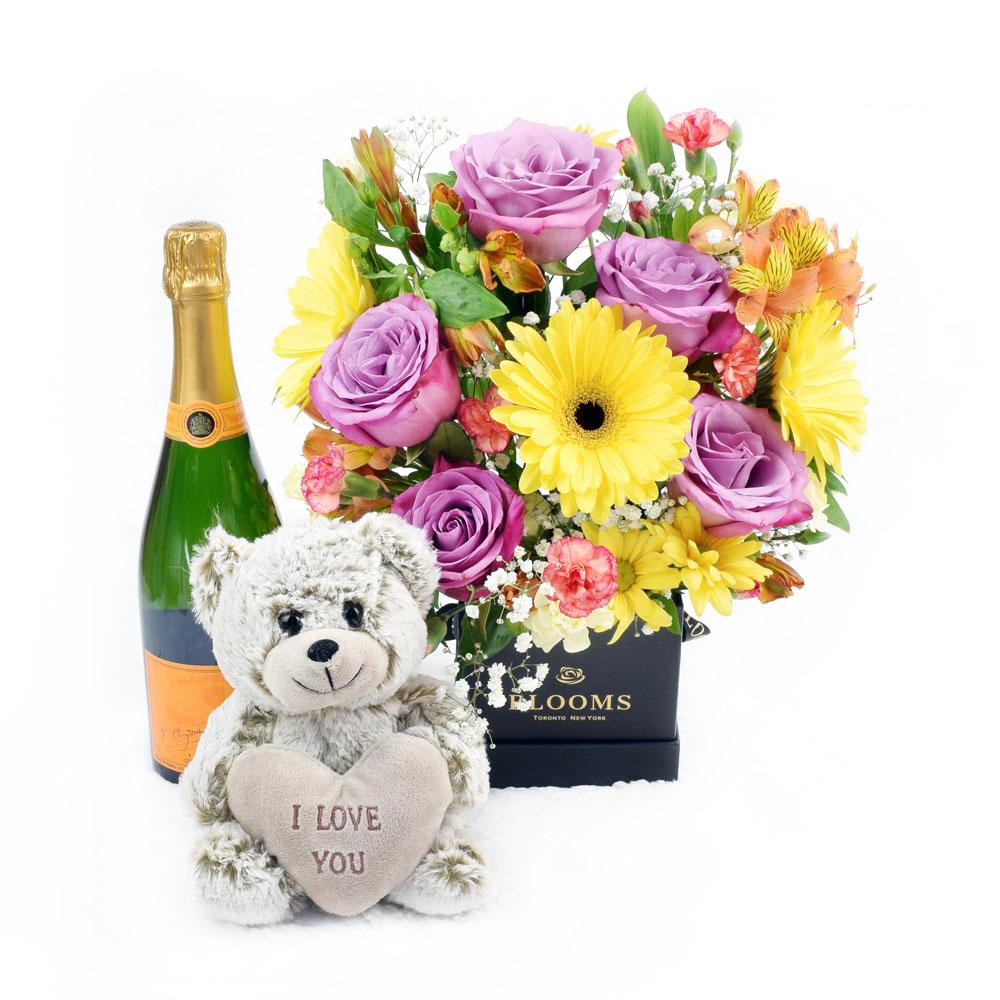The image features a professionally arranged Valentine's or romantic gift set on a white background. At the forefront sits a small, light gray teddy bear holding a heart that reads "I LOVE YOU" in all caps. Directly behind the bear, to the left, is a green bottle clearly identifiable as champagne, adorned with gold foil at the top and a wraparound label that's partly orange and blue. To the right of the bear is a vibrant bouquet of mixed flowers, including purple roses, yellow sunflowers, pink flowers, and white lilies, accented with lush green foliage. The bouquet is elegantly contained within a black box labeled "BLOOMS." Together, these items create an alluring and heartfelt gift ensemble.